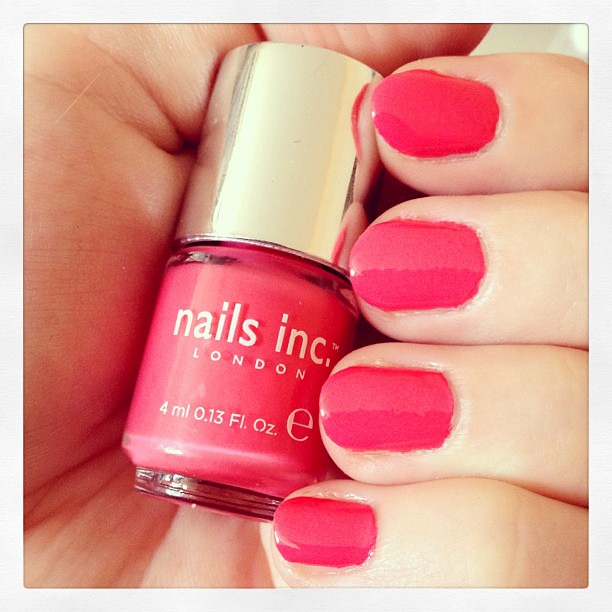This square close-up image features a small hand—presumed to be a woman's—holding a bottle of Nails Inc. London nail polish. The nail polish bottle has a gold cylindrical cap and a glass base. The label on the bottle also reads "4 milliliters, 0.13 fluid ounces." The nail polish color is a dark pink, almost a light red, which matches the polish on the hand's fingernails. The fingers, shown on the right side of the image, appear freshly painted with neat, glossy coats, giving a polished and well-manicured look. The image has a thin white border, adding a clean frame to the composition.